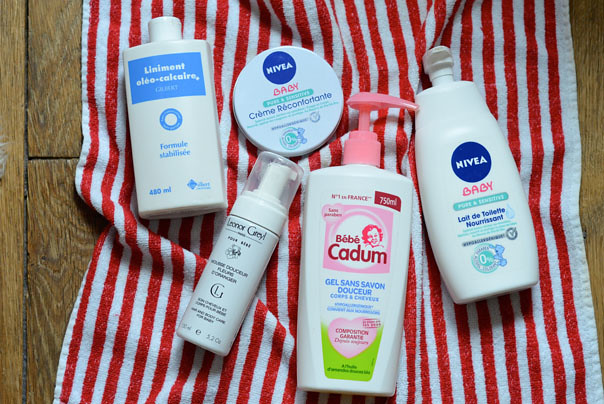This photograph features an assortment of baby lotion products meticulously arranged on a brown wooden surface. These products rest atop a peppermint-striped towel adorned with striking red and white stripes, which enhances the visual appeal of the display.

1. **Far Right**: The first product is a bottle labeled "Nevaeh Baby." While the exact text is challenging to decipher due to its small size, it is identifiable as a baby lotion.
   
2. **Bottom Left of the Nevaeh Baby Lotion**: Here, you find a pink product labeled "Baby Kodam." This product features an image of a baby on its front, underlining its target demographic.
   
3. **Top Left of the Baby Kodam Lotion**: Another "Nevaeh Baby" product is positioned here, labeled "Creme RÉfection," suggesting it may have French origins or influence.

4. **Bottom Left of the Nevaeh Baby Creme**: A spray bottle is visible, which appears to be either sunscreen or a tanning oil spray.

5. **Top Left of the Spray Bottle**: The final product looks like an ointment, potentially a liniment or something similar with the label hinting at the term "Calcareum." 

Overall, this ensemble of five baby care products creates an organized and visually coherent presentation, set against the inviting, warm tones of the wooden surface and the vibrant, striped design of the towel underneath.